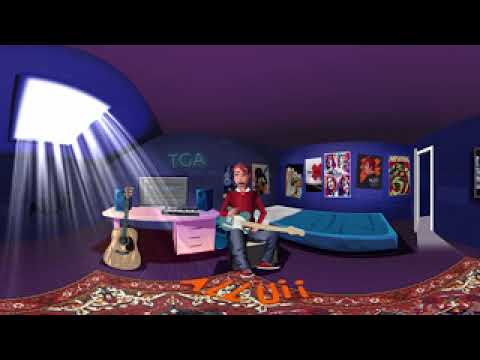This horizontally aligned rectangular image appears to be an animated or cartoon illustration of a young man sitting in his bedroom, holding a blue and white electric guitar on his lap. The young man, who has short brown hair, is dressed in a red long sleeve shirt, gray pants (or jeans), and red sneakers. Despite being slightly blurry, his open mouth is still discernible. He is seated in front of a bed that is covered with a blue blanket and a white sheet.

The bedroom walls are primarily blue, with a purple ceiling. On the left side of the image, a large window with sunlight streaming through it casts rays of light into the room. The sunlight highlights part of the blue wall and a white square. Below this window, there's a white or pink desk with a monitor and keyboard. Leaning against the desk is a brown acoustic guitar.

Adorning the blue wall behind the young man are the capital letters "TGA" in bright neon green, along with numerous posters. To the far right of the image, there is an open door with white molding, and beneath the young man, there appears to be a red and white carpet. This animated setting creates a vibrant and visually engaging scene that captures the essence of a musician's personal space.